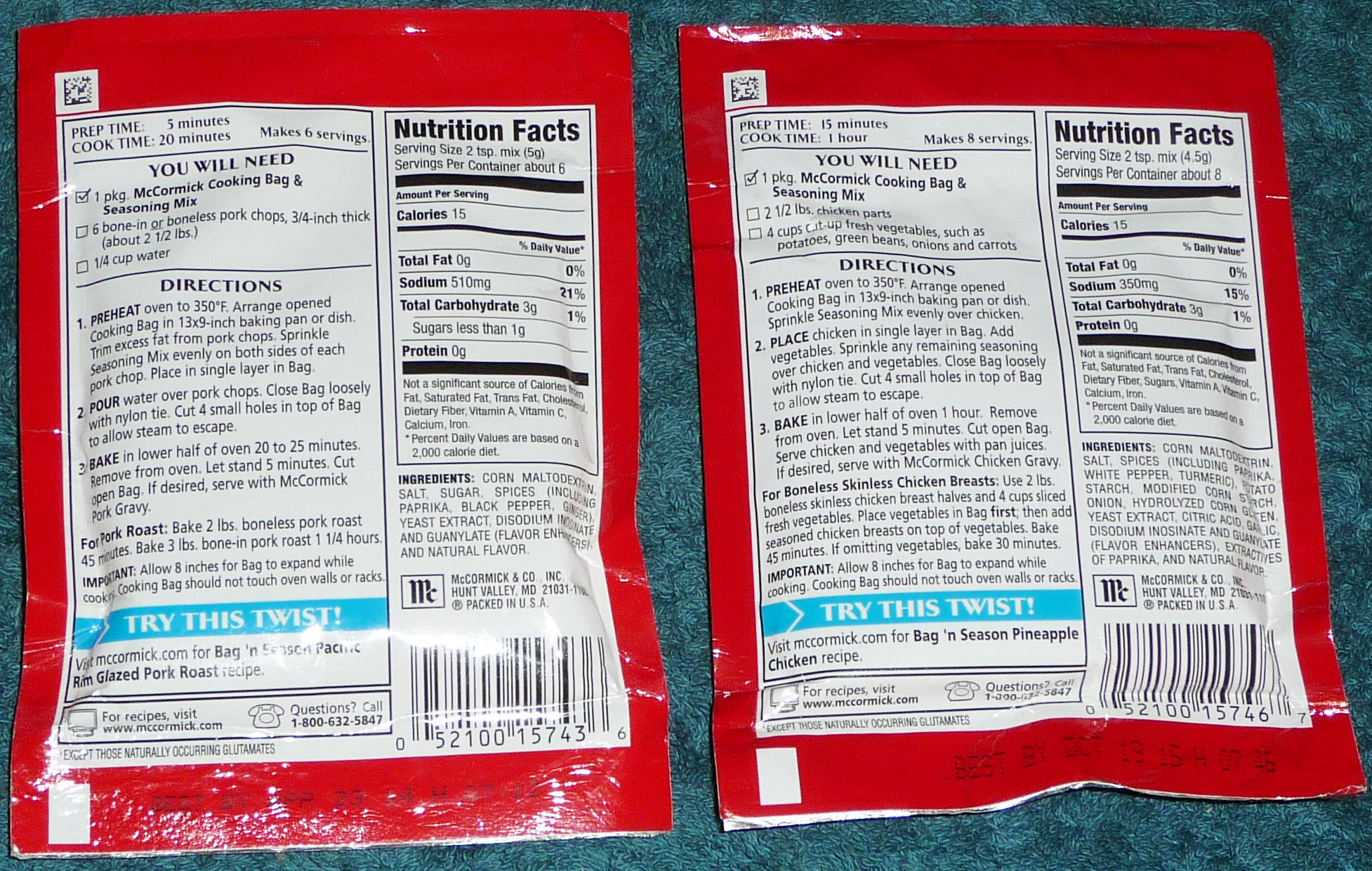The image depicts the back of two red packages, likely for seasoning mixes or similar cooking products, lying face-up on a greenish-blue surface, possibly a counter or carpet. Each package features a prominent white section containing directions and nutrition facts. The packages differ in preparation and cooking times, with one stating 5 minutes of prep and 20 minutes of cooking, while the other requires 15 minutes of prep and 1 hour of cooking. Both packages are from McCormick, as evidenced by the logo visible near the barcodes in the bottom right-hand corner. The text details the ingredients needed: one McCormick cooking bag and seasoning mix, six pork chops (either bone-in or boneless), and 1¼ cups of water. Directions also include preheating instructions and tips for a twist on the recipe. The information is printed in black on the white background, with nutrition facts segmented within the white area.